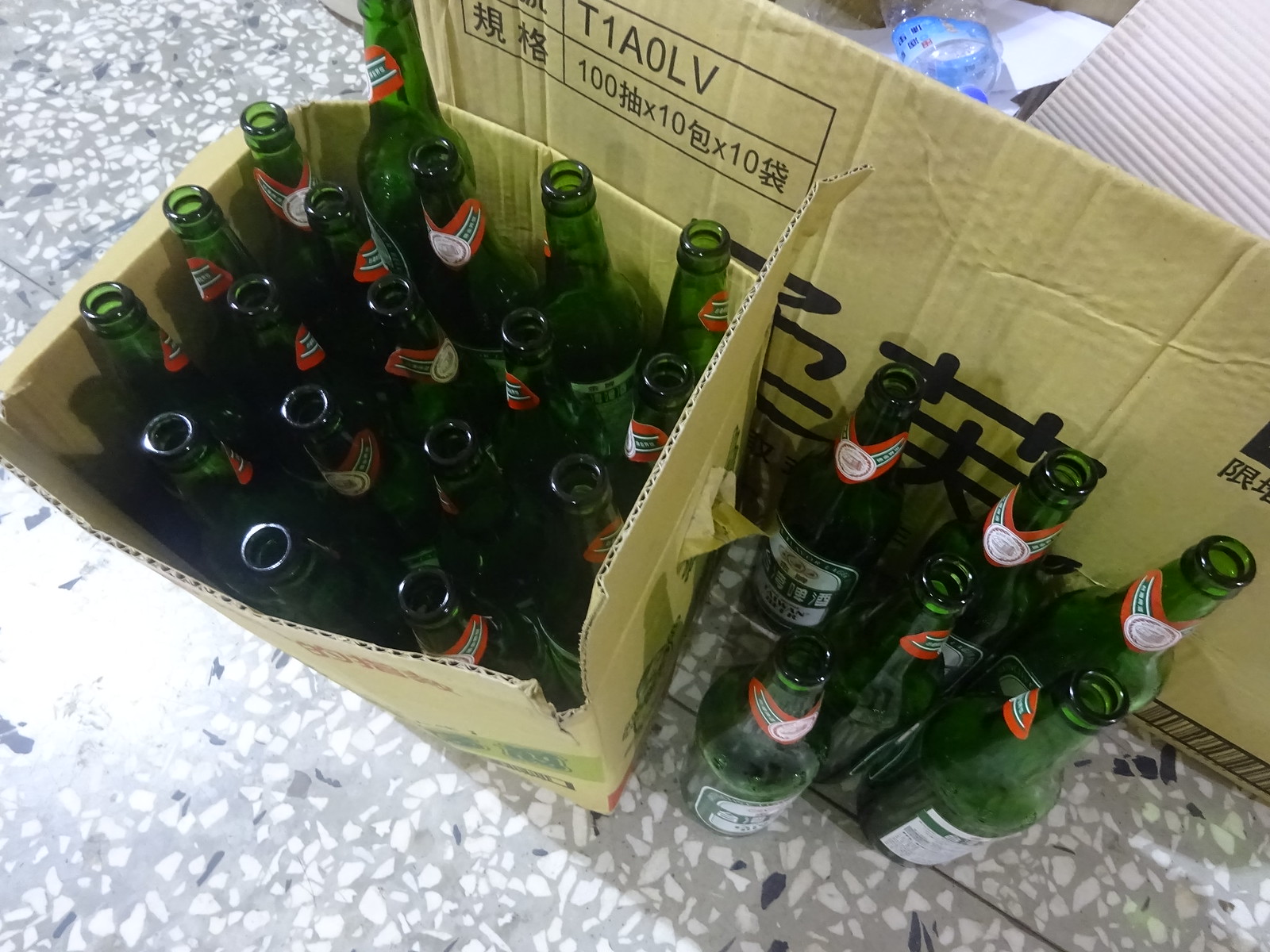This close-up color photo features a light gray linoleum floor with white and dark gray specks resembling rocks. Centered in the image are two cardboard boxes. The box on the left is open and contains approximately 21 empty green bottles, each adorned with a red label with black writing and another label around the neck, suggesting they may have held beer. To the right of this box, six identical empty green bottles stand upright. Behind this scene, a larger cardboard box with Japanese or Chinese writing on it appears. This box seems to serve as a recycling bin and is filled with white corrugated cardboard material, paper, and possibly an empty water bottle.